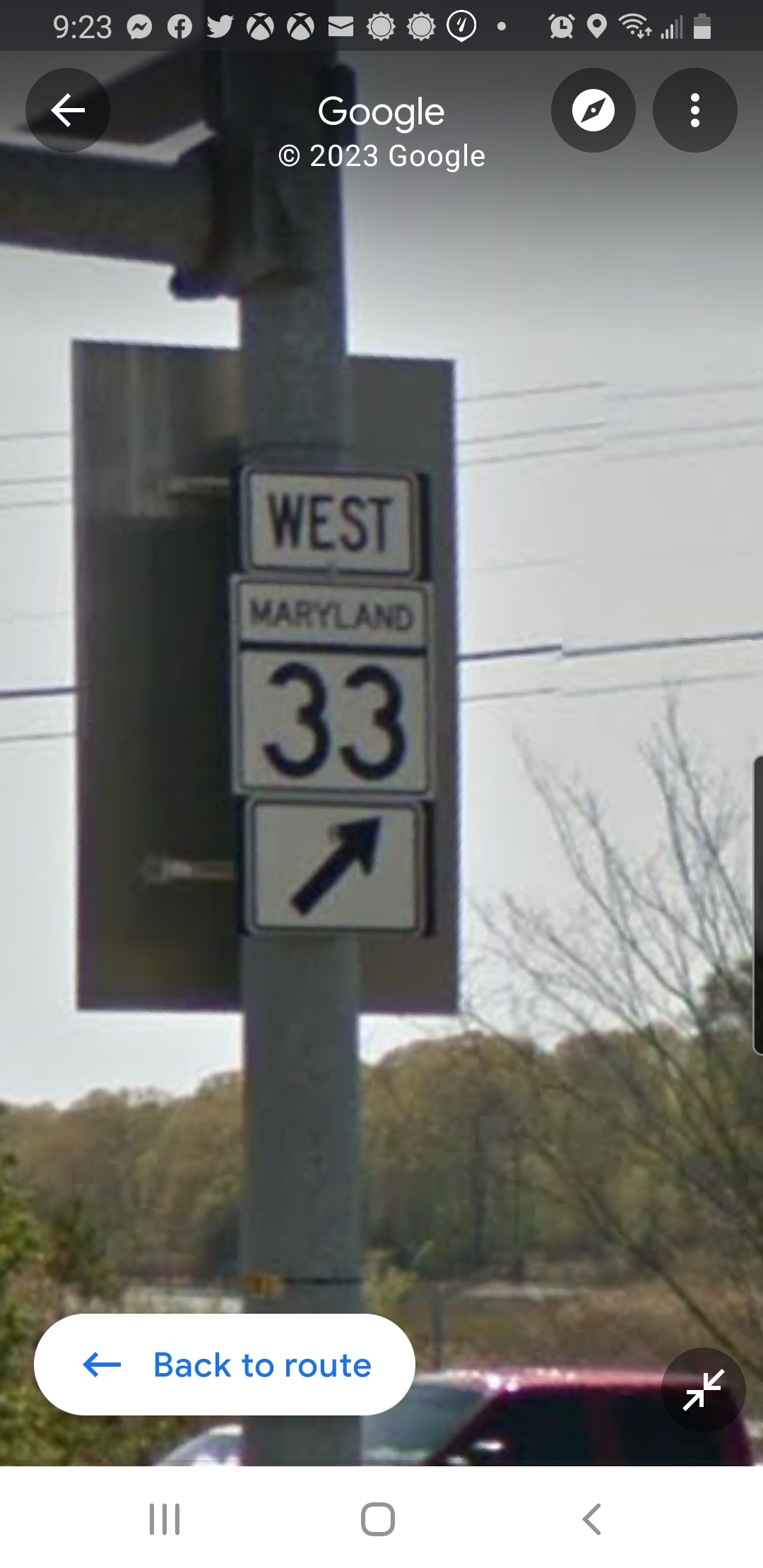This image is a screenshot from an Android phone, with the status bar showing various icons and notifications at the top. The time displayed is 9:23 AM, in white text on a translucent dark gray background. The top left corner features a white arrow pointing left, indicating a back function. The top middle of the screen displays "Google" in white text, followed by a copyright symbol and "2023 Google." Additionally, there are two round icons, likely a compass and a menu represented by three dots.

The main content of the screenshot is a Google Street View image featuring a large, metal gray pole slightly offset to the left. The pole displays a series of white signs with black text: at the top is a rectangular sign reading "West," followed by a square sign that says "MARYLAND" in all caps with the number "33" beneath it. Below these, a small square sign has a black arrow pointing diagonally from the top left to the top right. Near the bottom left of the image, there's a white pill-shaped button with blue text that says "Back to Root," accompanied by a blue arrow pointing left.

In the background, there are light green trees and a grassy area with hints of light brown, suggesting a seasonal change. The top of a maroon truck and a white car are visible in the lower part of the image. The screenshot includes several phone notifications, such as from Facebook, Twitter, Xbox Live, Yahoo! Email, and Weather, along with indicators for Wi-Fi signal, battery level at 60%, and an alarm.